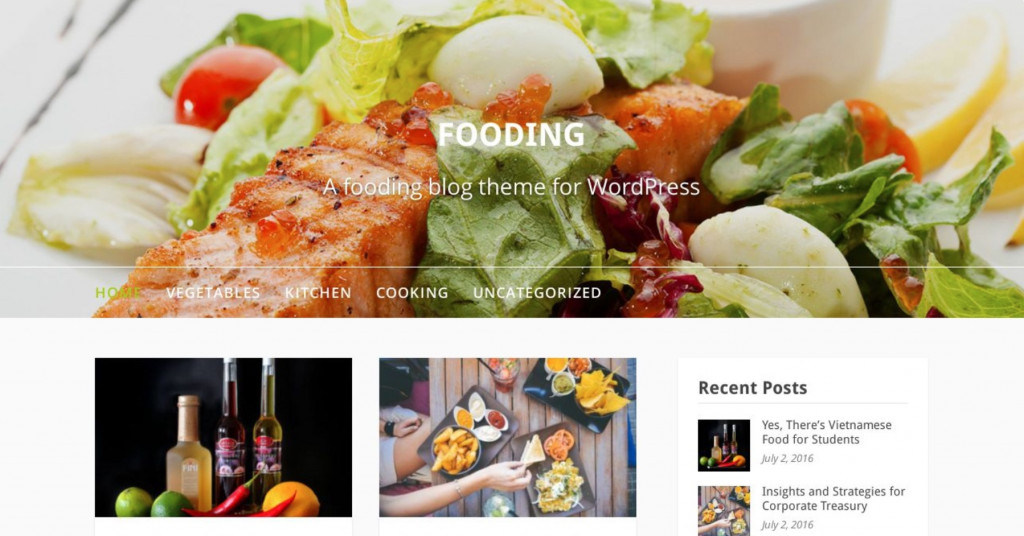An inviting food blog showcases an array of vibrant and healthy dishes, styled to perfection. The blog's header prominently features the word "Fooding" in white, set against a backdrop of diverse, nutritious foods. Central to the imagery is a plate teeming with fresh green lettuce, succulent salmon, perfectly hard-boiled eggs, and bright cherry tomatoes, all accompanied by a refreshing lime wedge on the right.

Additionally, the page navigation is crisp and user-friendly, denoted by green-highlighted 'Home' and other white-labeled sections like 'Vegetable Kitchen,' 'Cooking,' and 'Uncategorized.' The home page displays a well-composed collage below the header. On the left, it features an image of dressing contained in two elegant wine bottles, flanked by vibrant lime wedges, chili peppers, and an orange. Nearby, a table spread entices with dishes of finger foods—chips paired with assorted salsas and guacamole, sliced tomatoes, and dipping sauces alongside potato wedges. Hints of social interaction are visible as arms reach for the delightful fare.

On the right side of the page, some recent posts are summarized with thumbnails and titles. Among them, articles spotlight "Yes, There's Vietnamese Food for Students" and "Insights and Strategies for Corporate Treasury," complete with publication dates, offering a glimpse into the diverse content available on this meticulously curated food blog.